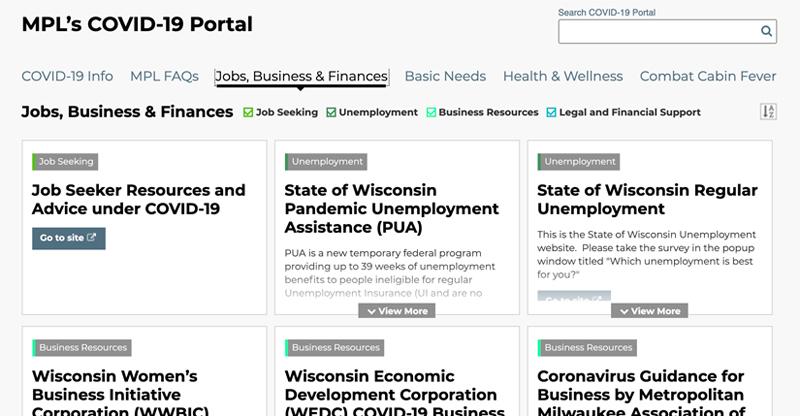This is a detailed screenshot of the MPL COVID-19 Portal website. The top left section prominently displays the text "MPL's COVID-19 Portal" in black. Just to the right of this title, there is a search bar labeled "Search COVID-19 Portal" situated above it. Below the portal title and search bar is a navigation menu featuring six links: "COVID-19 Info," "MPL FAQs," "Jobs, Business, and Finances," "Basic Needs," "Health and Wellness," and "Combat Cabin Fever."

Further down, the section titled "Jobs, Businesses, and Finances" can be seen, accompanied by four checkboxes labeled "Job Seeking," "Unemployment," "Business Resources," and "Legal and Financial Support." Below the checkboxes, there is a three-column grid displaying articles, with two visible rows of content, providing a structured and accessible layout of relevant information.